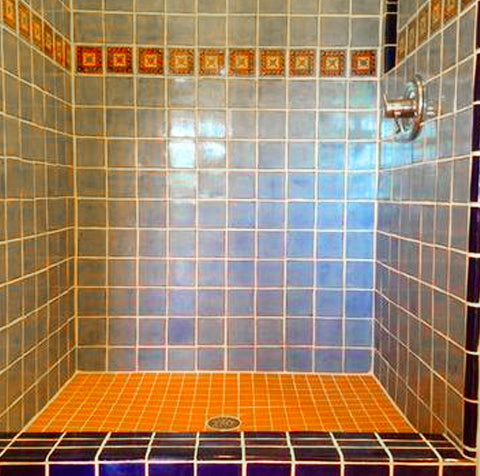The image depicts the interior of a square shower stall with a striking tiled design. The floor is covered with small orange tiles, while the entrance step-over is adorned with larger cobalt blue tiles. The interior walls are predominantly light blue, likely affected by the room's lighting, and feature a distinct patterned strip with an "X" inside a box, suggesting a Spanish motif. This patterned strip runs above the modern temperature control, which consists of a sleek straight lever on the right side. Additionally, there's a dark blue outline on the right edge and around an indented shelf for toiletries situated above the water control. Notably, a few red tiles with symbols decorate the top of the shower, and the floor includes a central drain. The stall is open with no curtain visible.